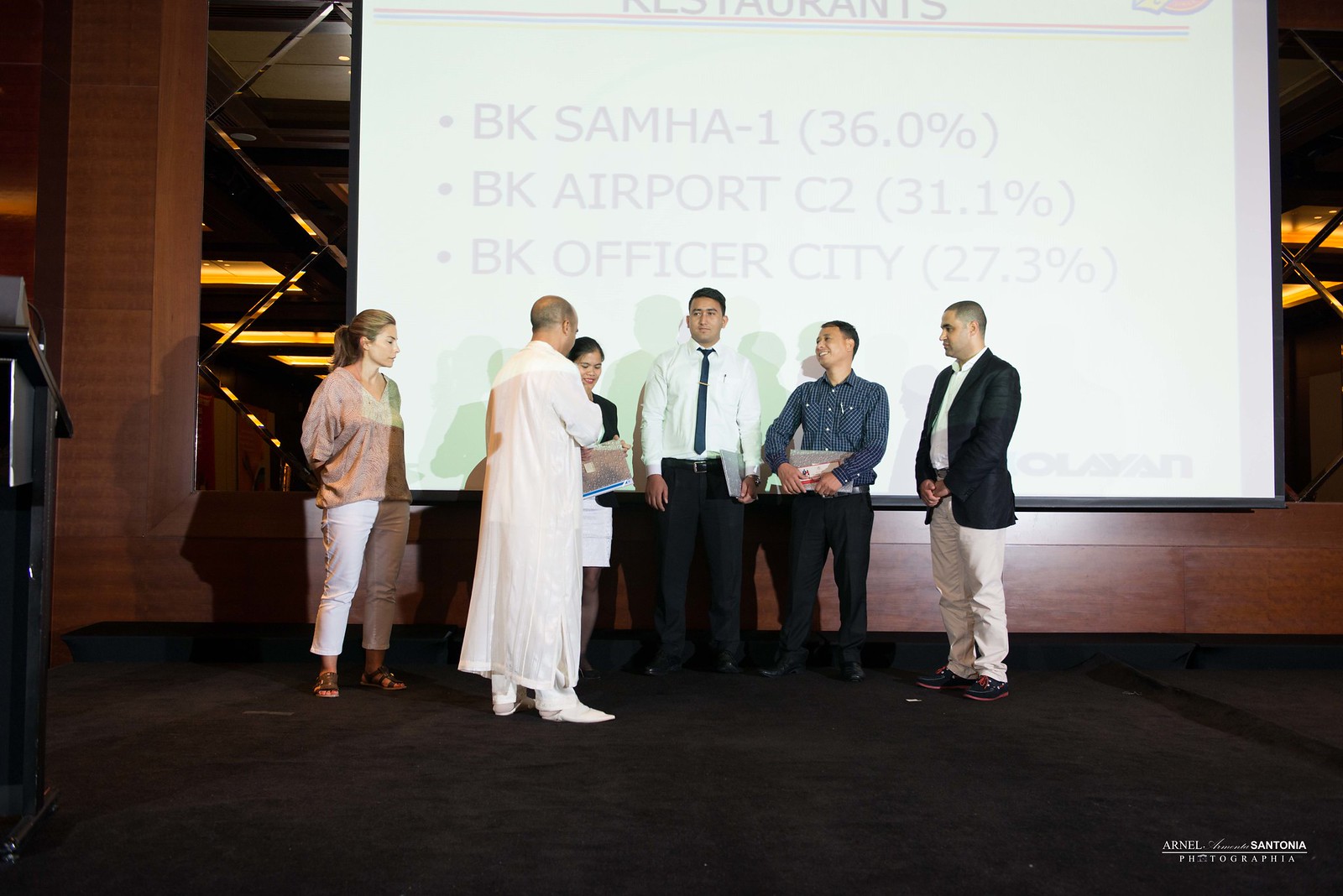The photograph captures six individuals standing in front of a large, partially visible projection screen set against a backdrop that includes light brown wooden walls adorned with diamond-patterned mirrors on the left. The screen, slightly off-center to the right and wider than it is tall, displays a faint green PowerPoint slide with black text reading, "BK SAMHA-1 36.0%, BK Airport C2 31.1%, BK Officer City 27.3%." The group consists of four men and two women positioned on a black carpeted floor. Prominently, a man in a long white robe, white pants, and white shoes appears to be handing out items to the others. The exact nature of these items is unclear. The background behind the screen includes indistinct features such as a glass-like backing, a pillar on the left, some lighting, and possibly steps, giving a sense of depth and context to the gathering area.